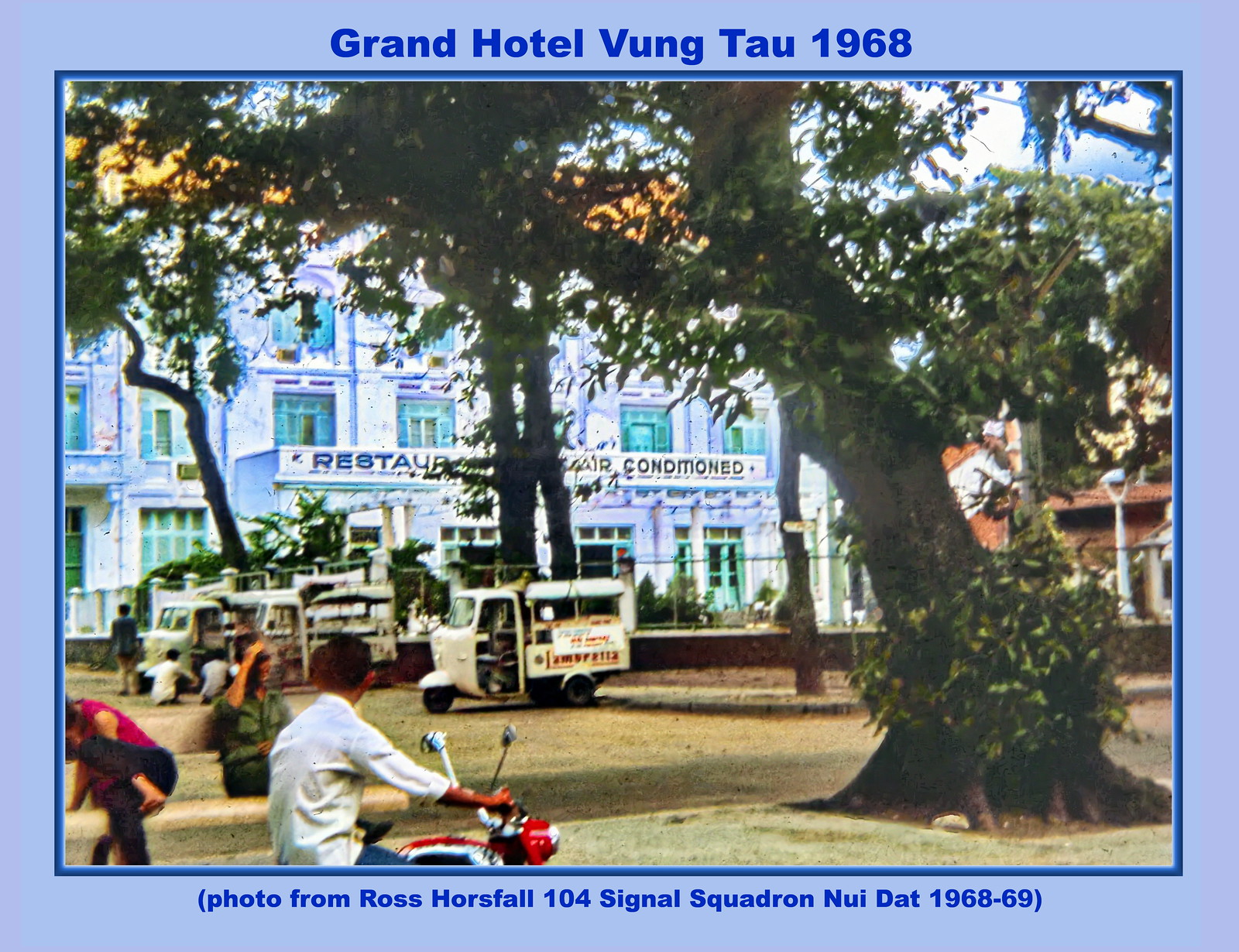The photograph, titled "Grand Hotel, Vung Tau, 1968," shows a lively scene during the Vietnam War era. Dominating the background is a large, possibly three or four-story hotel building, appearing bluish due to the image's vintage coloring. The hotel features signs that read "Restaurant" and "Air-Conditioned." In the foreground, a young man wearing a long-sleeved white shirt rides a small, red moped, facing away from the camera. To the right of this scene, a barefoot woman sits on a park bench next to a man with a cap shielding his eyes. The setting is likely a downtown market square, evidenced by the presence of food trucks, three in a row, and various white vehicles parked along a fence near the hotel. Tall trees, with prominent trunks and various green leaves, are scattered around, adding to the open, airy feel of the location. The photograph includes a caption that reads, "Photo from Ross Horsfall, 104 Signal Squadron, Nui Dat, 1968-69."